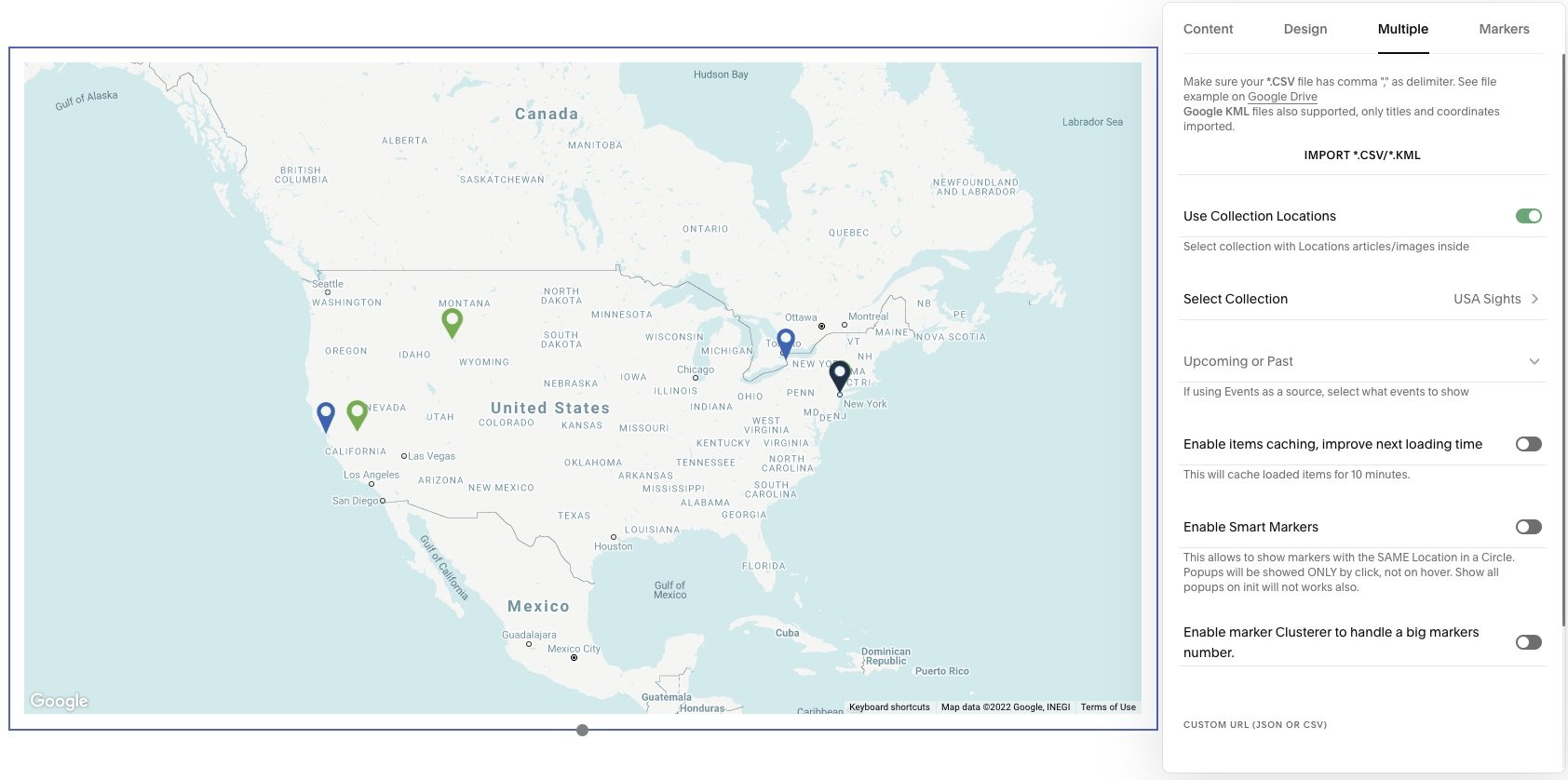This image is from a webpage featuring a map that includes the United States, most of Mexico, and a significant portion of Canada. The countries are depicted in a very light gray color, while surrounding bodies of water such as the oceans, the Gulf of Mexico, the Great Lakes, and other waterways are illustrated in a very light sky-blue hue. The map's text, which labels various regions, is presented in a light blue font that is somewhat difficult to read.

At the center of the map, directly above Colorado and Kansas, "UNITED STATES" is inscribed in capital letters. Each U.S. state is also labeled in this faint blue, capital-letter font. Similarly, the map marks the visible Canadian provinces and most of Mexico, extending to include parts of Guatemala and Honduras.

Additionally, the map features teardrop-shaped markers indicating specific locations: a blue marker in California, another in Nevada, a green marker in Montana, and two blue markers in New York and New York City.

On the right-hand side of the image, there are instructions under the headlines "Content," "Design," "Multiple," and "Markers." The instructions include a note about ensuring that your CSV file uses commas as delimiters, providing guidance on how to import your CSV file effectively.